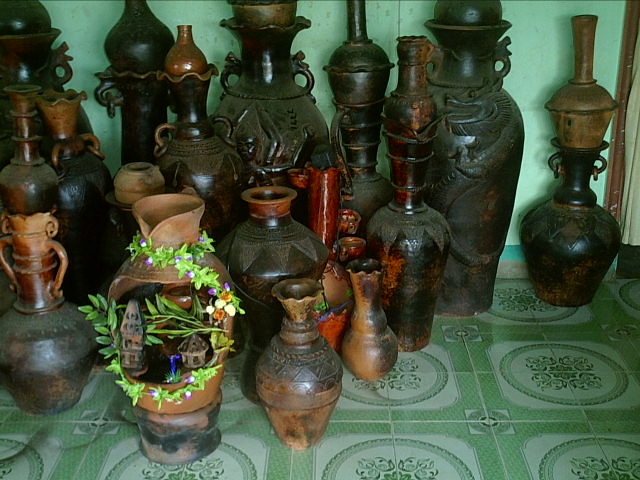This colorful landscape photo captures a collection of intricately designed jars, vases, and bowls standing on a detailed green and white tiled ceramic floor. The tiles exhibit a pattern of green squares punctuated by circular floral designs at their intersections, lending an artistic touch to the floor. The back wall is painted a lively lime green, adding a vibrant backdrop to the scene. The array of ceramics, which appear predominantly in dark shades of brown, black, and dark grey, are carefully arranged against one side of the room. Each piece stands vertically, resembling urns or large jars, some adorned with intricate carvings while others remain plain. Many of the jars feature two small handles near the neck, enhancing their traditional appearance. Of particular interest is a jar positioned towards the front left; it has been cut open and reveals a charming diorama inside, decorated with faux green ivy and leaves, contrasting beautifully with its dark and lighter brown hues. The collective arrangement of these ceramics creates a visually rich and harmonious composition.